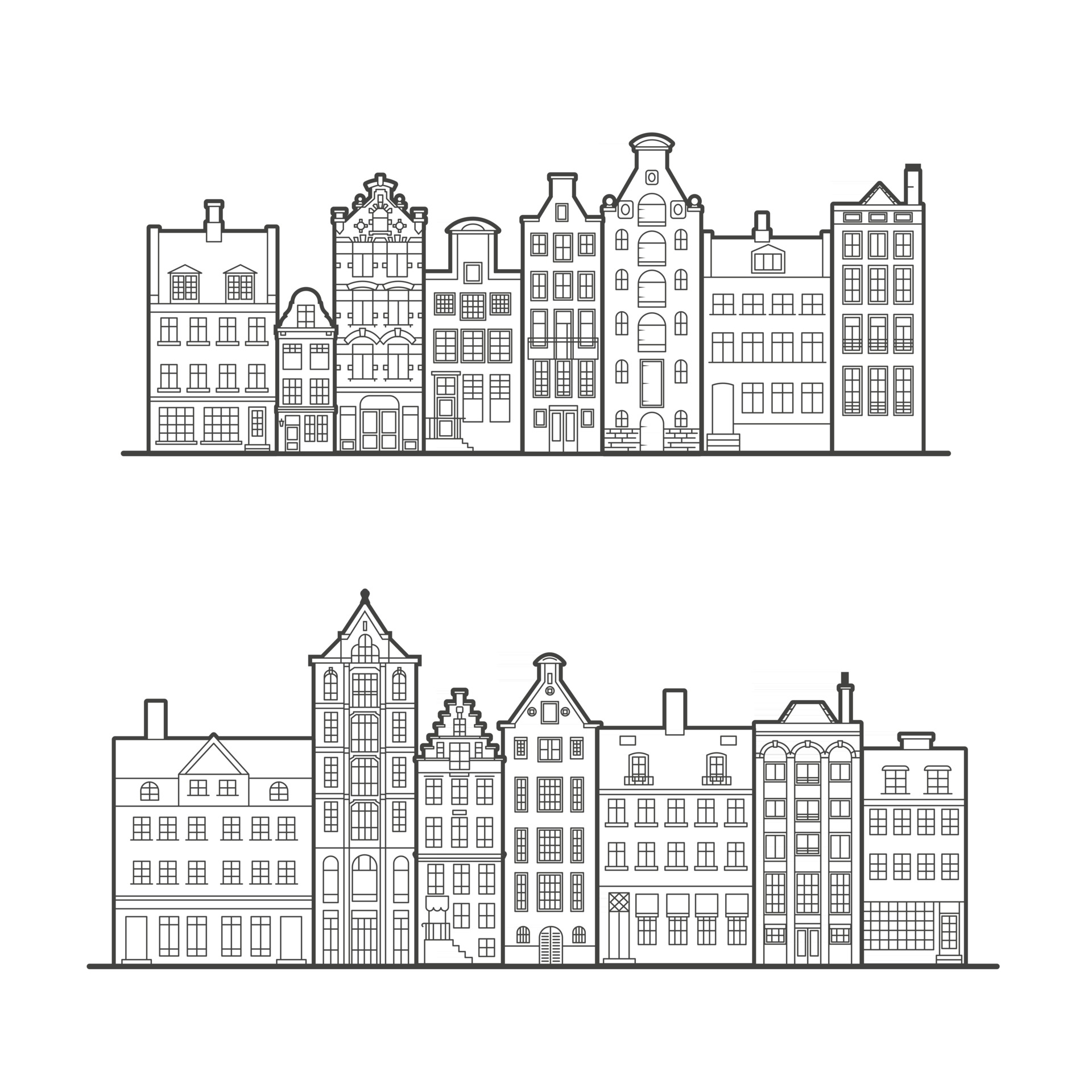This black and white pen and ink drawing is comprised of two vertically stacked images, each depicting a row of city buildings reminiscent of brownstones. The buildings in both rows are tall and narrow, ranging from four to five stories high, and exhibit differing heights, widths, and architectural details. The top image showcases eight buildings, while the bottom features seven, each adorned with varying styles of windows, doors, and some with chimneys. All the buildings are intricately detailed, emphasizing their uniqueness, and are flanked by a black border at the bottom of each drawing. The illustration captures the essence of a city block with its diverse yet cohesive multi-story structures, presented in a stark, black and white format without any text or color elements.